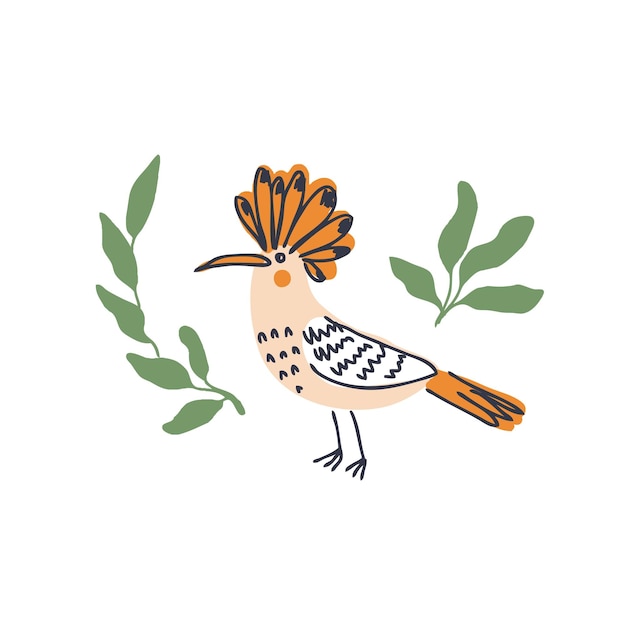The image portrays a simple, hand-drawn and possibly marker-based bird in a folk art style, primarily using light pastel colors. The bird has a tannish pink base with distinctive orange features, including its comb feathers, tail feathers, beak, and a round cheek patch. The wing is white with gray squiggles, and the bird stands on skinny legs with webbed feet, highlighted by minimal line work defining the beak, feathers, tail, and wing. Surrounding the bird are two sets of green leaves: one set with six leaves on the left and another with four leaves on the right. The overall design is clean and minimalist, set against a stark white background, emphasizing its quaint and artistic simplicity.